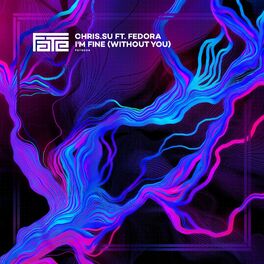This detailed album cover for Chris Su featuring Fedora is titled "I'm Fine (Without You)." Positioned in the top left-hand corner, the title and the accompanying text are rendered in white, alongside a distinct logo or symbol. The background is a lavish tableau of abstract art, characterized by a chaotic mix of colors with no discernible pattern, giving an impression as if paint has been spilled freely. This artwork features flowing strands and rivers of color, including various shades of blue—dark blue, light blue, and indigo—along with vibrant purple, pink, and fuchsia hues. The fuchsia coloring is dynamic, evoking the appearance of electricity or lightning. All these elements are set against a dark, purplish-black backdrop. Additionally, there's a colorful border around the square album cover, with alternating shades of hot pink, electric blue, teal, and purple, adding to the vibrant and eclectic aesthetic. Some smaller, unreadable text is also present on the cover.